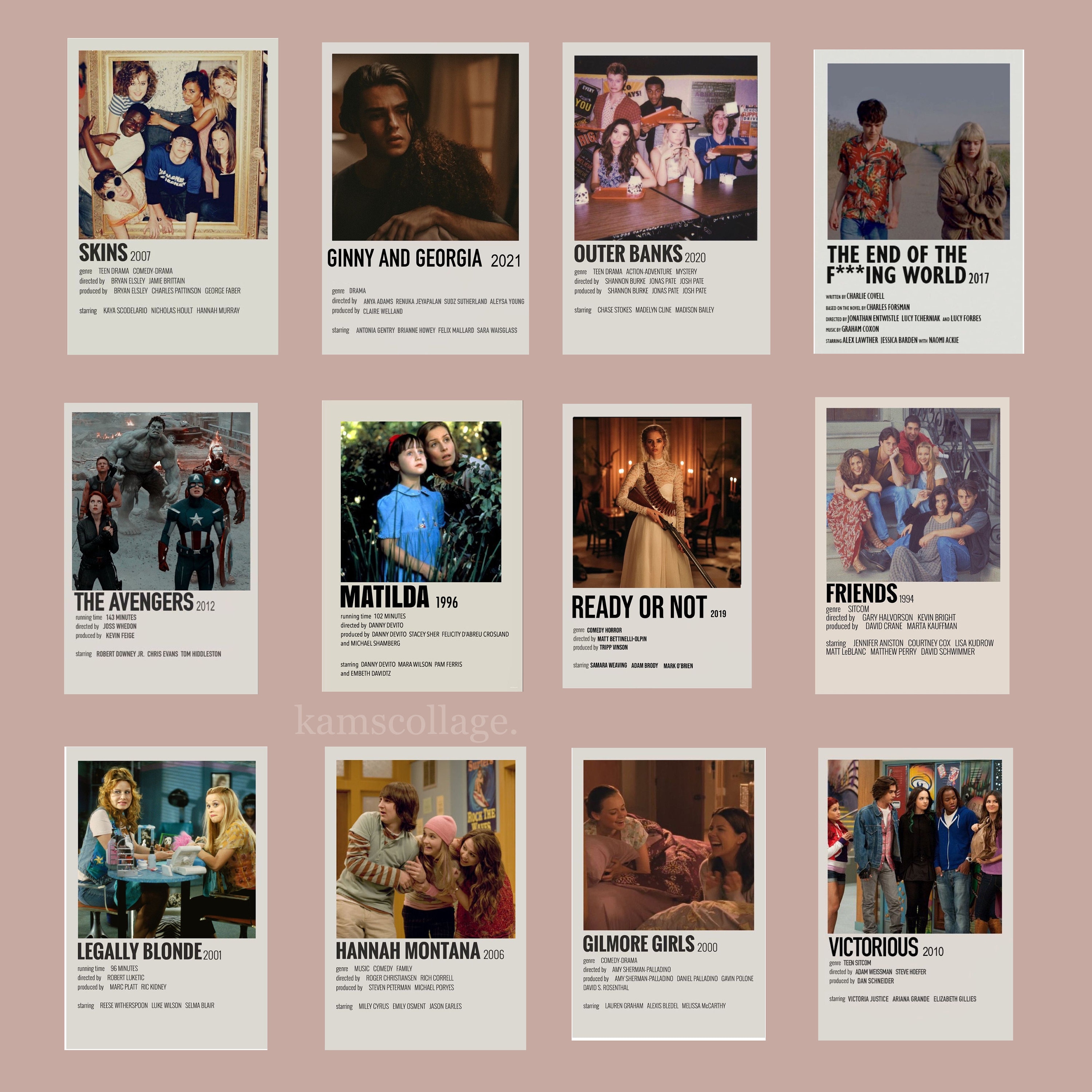Set against a pink background, this detailed collage displays twelve Polaroid-like images arranged in a 4x3 grid, each representing a different TV show or movie. Each Polaroid features a distinct scene, title, and an illegible description in small font. The top left image captures a scene from "Skins," showcasing several characters looking through a picture frame. To its right is "Ginny & Georgia 2021," depicting a person in a dark image wearing a black shirt. Next is "Outer Banks," illustrating people gathered around a table, followed by a scene from "The End of the F***ing World," featuring a boy and girl walking down a street.

In the second row, the leftmost image is "The Avengers," showing the superhero team amidst rubble. Next, "Matilda" portrays Matilda and a woman gazing into the distance. The following image is from "Ready or Not," with a woman in a wedding dress holding a rifle pointed downward. The last image in this row captures the iconic "Friends" cast sitting on a stoop.

The bottom row starts with "Legally Blonde," showing Reese Witherspoon and another actress at a manicure table. Next is "Hannah Montana," featuring three actors looking to their right while holding onto each other. Following is "Gilmore Girls," with two girls laughing in a bed, and the final Polaroid displays "Victorious," presenting five characters looking off to the side.